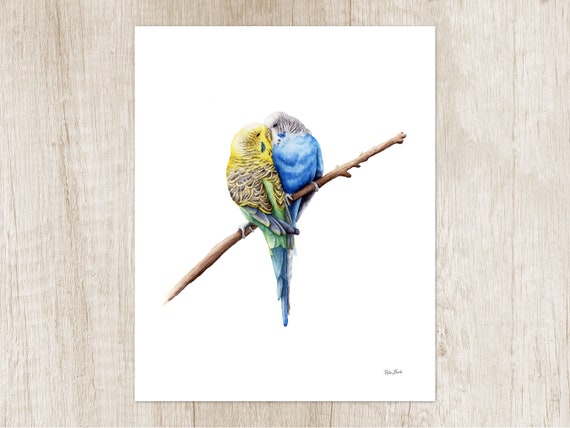The image displays a vivid painting mounted on a beige beechwood-textured wall, showcasing a lively scene of two colorful parrots perched on a slender, brown branch that stretches diagonally from the lower left to the upper right. The bird on the left features a bright yellow head, a vibrant greenish-brown body, and blue tail feathers. It looks toward the right, where it faces the second parrot, which has a muted gray head transitioning into a striking blue body and tail. The birds appear to be engaged in a close, intimate moment with their beaks almost touching, as if they are kissing. The background of the painting is white, emphasizing the colorful details of the parrots. The painting is square and there is a small signature located in the bottom right corner, possibly indicating the artist's initials. The wooden wall behind the painting has slots that add to its rustic charm.